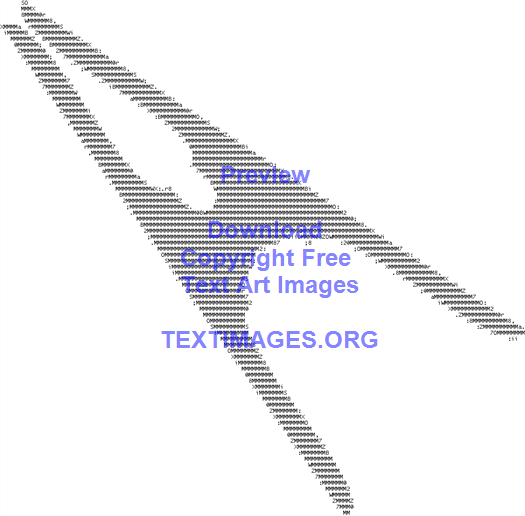The image features a central object resembling a clothespin or safety pin composed of intricate black and gray components, possibly small screws or nails. The object is angled to the top left against a pristine white background, emphasizing its detailed construction. Cascading across the image in purply-blue and light blue lettering are the words: "PREVIEW," with a bit of space followed by "DOWNLOAD," and directly below, "COPYRIGHT FREE." Beneath these lines, in darker blue text, "TEXT" is prominently displayed, followed by "ARTIMAGES" in a lighter shade. Continuing below this, in light blue text, it reads "TEXTIMAGES.ORG."